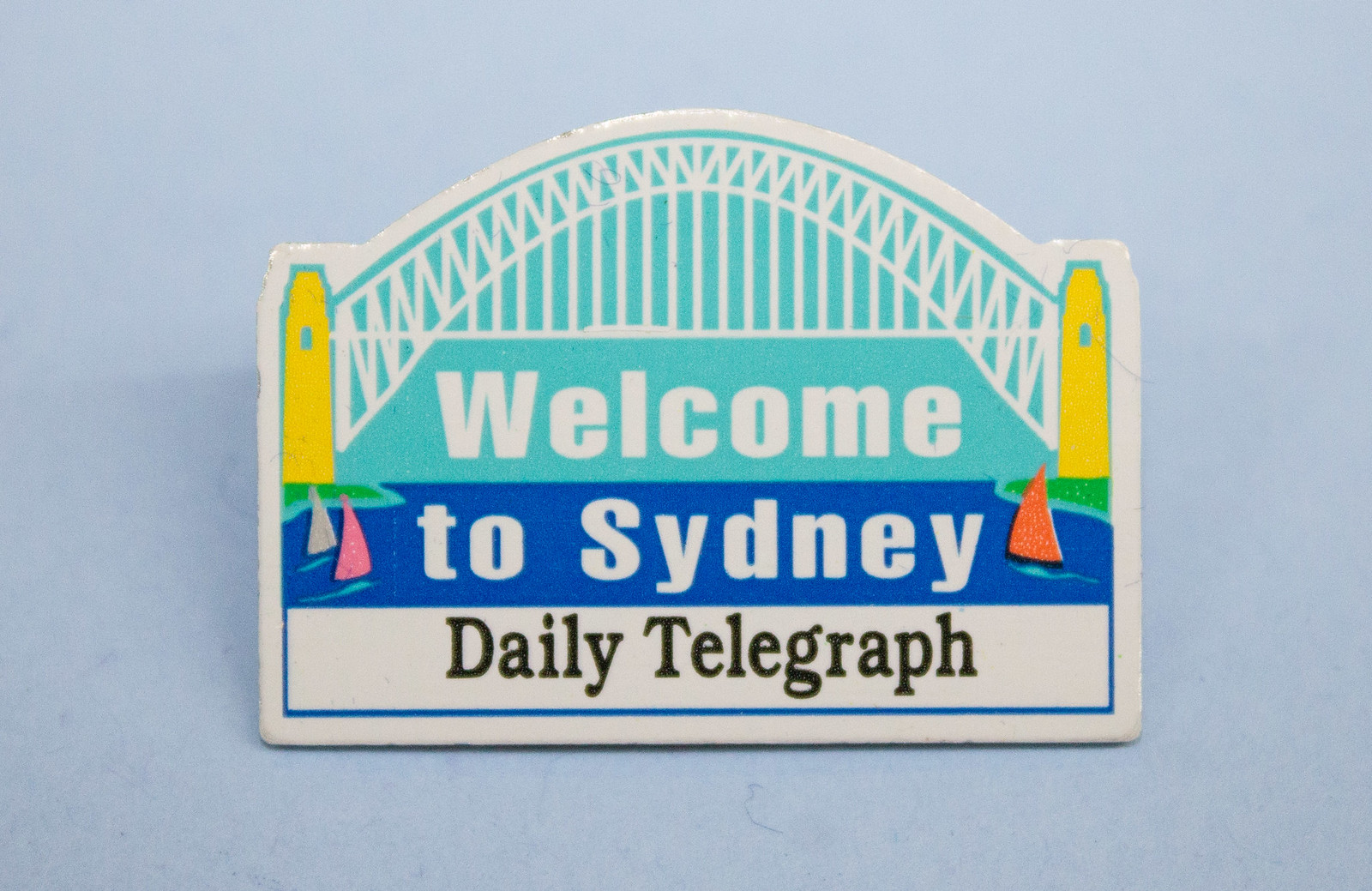This photograph is of a small, colorful sign, possibly a pin or desk sign, featuring a detailed cartoon drawing. The sign has a vibrant illustration of a bridge with yellow towers on either end and white lines forming an arch. Below the bridge, a blue strip represents water, adorned with three small sailboats with sails in gray, pink, and orange. The text on the sign is arranged in three segments: "Welcome" in white text on a light blue background below the bridge, "to Sydney" on the blue water strip, and "Daily Telegraph" in black print on a white strip at the bottom. The overall background of the photograph is plain, highlighting only the sign without any other elements or people visible, and the sign is placed on a blue surface.